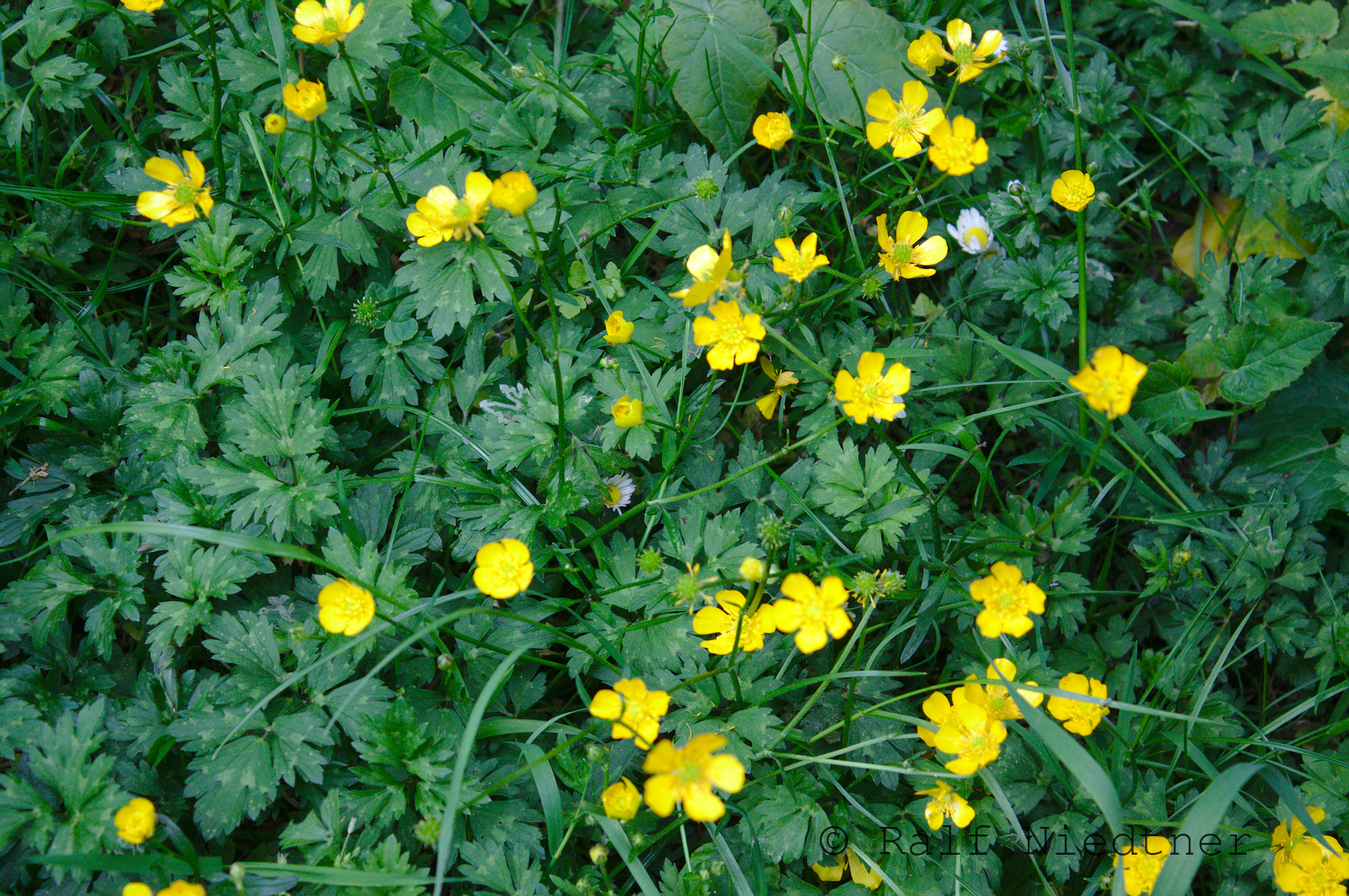This photograph captures a lush, unmanicured patch of wild vegetation, likely in someone's yard or in a random countryside location. The scene is dominated by an array of green leaves, many resembling cilantro but not actually being cilantro, with some heart-shaped leaves that might be mistaken for poison ivy. Scattered amidst this verdant expanse are over 20 to 30 yellow flowers, each with four petals, and there are also hints of white and yellow buds. It appears there may be dandelions and other unidentified wildflowers amongst the mix. The dense foliage creates dark, shaded areas within the brush, and a few grass shoots are visible. The atmosphere seems humid and damp, possibly indicating the photograph was taken after rain or in a tropical environment. A watermark on the bottom right corner credits Ralph Niedner as the photograph's author. The overall scene is abundant with natural, untamed beauty, captured in the daytime.